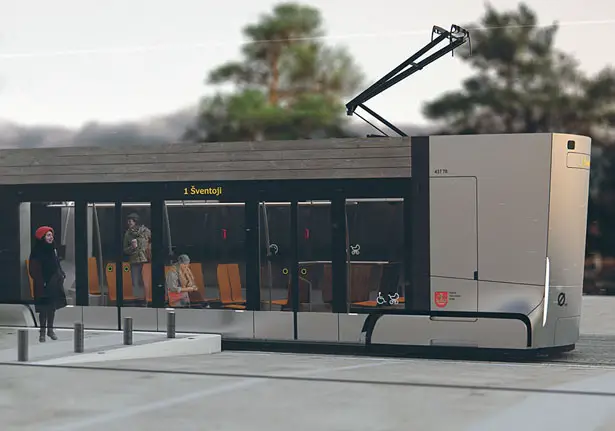The image depicts an outdoor scene featuring a meticulously crafted miniature train station with an electric streetcar, or tram, prominently displayed. The tram, which is sleek and metallic grey with black borders and large glass panels, stands at the station, connected to overhead cables by jointed black rods. Inside the tram, orange seats line the interior, occupied by passengers, while one person stands. The front of the tram is enclosed smoothly, giving it a modern, almost concept art-like appearance. The text "Sventagi" is written in yellow at the center of the tram. Outside on the platform, a woman dressed in a black coat, long pants, and a red beanie stands, adding a human touch to the scene. The background features green-leafed trees, a grey sky, and mountains to the left side, enhancing the realistic yet miniature setting.